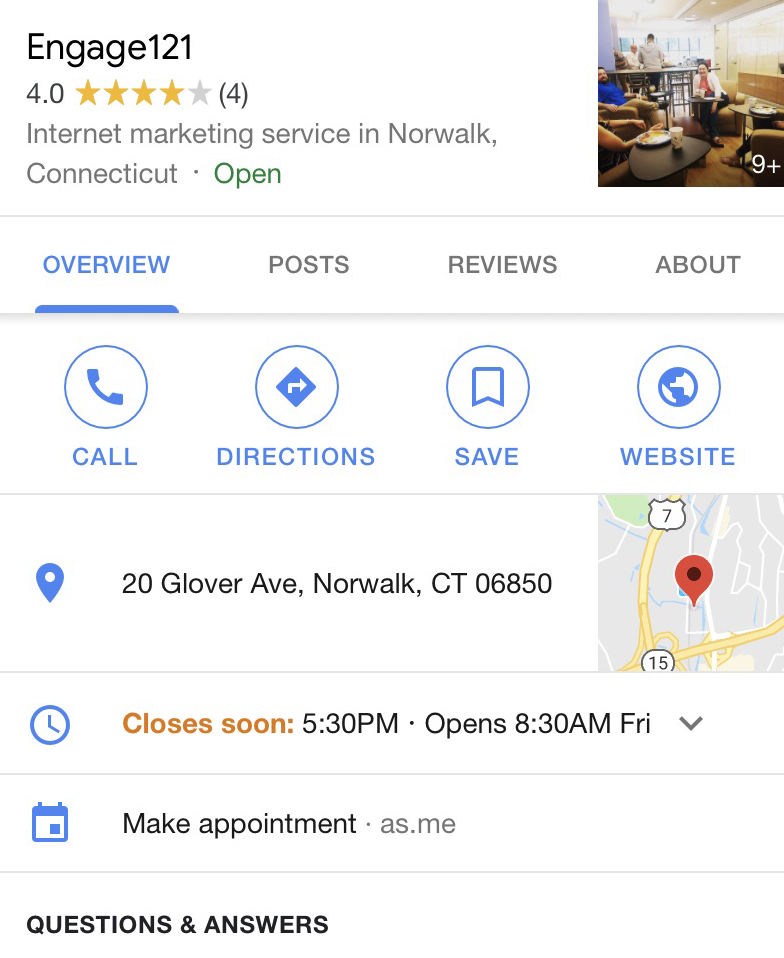**Descriptive Caption for Screenshot of Google Business Listing:**

The image is a screenshot taken from a phone displaying a Google business listing for "Engage121." The listing has a clean, white background with black text. In the upper left corner, the company name "Engage121" is displayed. To the right, there is a small photo of a man and a woman sitting in an office setting, looking at the camera.

Below the company name, the rating is shown as "4.0" along with four yellow stars and the note "4 reviews." In gray text beneath the rating, it states "Internet Marketing Service in Norwalk, Connecticut" and indicates that the business is currently open. 

The navigation menu includes blue and gray text with options such as "Overview," "Posts," "Reviews," and "About." Below these options, blue buttons are available for actions such as "Call," "Direction," "Save," and "Website."

A pin icon in blue marks the business address: "20 Clover Avenue, Norwalk, CT 06825," which corresponds to a Google Map on the right side of the screenshot marked with a red pin showing the location. Beneath the map, a green notice reads "Closing soon - 5:30 PM," and indicates that the shop opens at "8:30 AM." The current day is noted as "Friday."

Additionally, a blue calendar icon is next to a call-to-action that reads "Make an appointment," with a link provided as "as.me" in gray text. At the bottom left, a header "Questions and answers" appears in black text, indicating the conclusion of the displayed information. 

The screenshot ends here, showing a detailed overview of the Google business listing for Engage121.